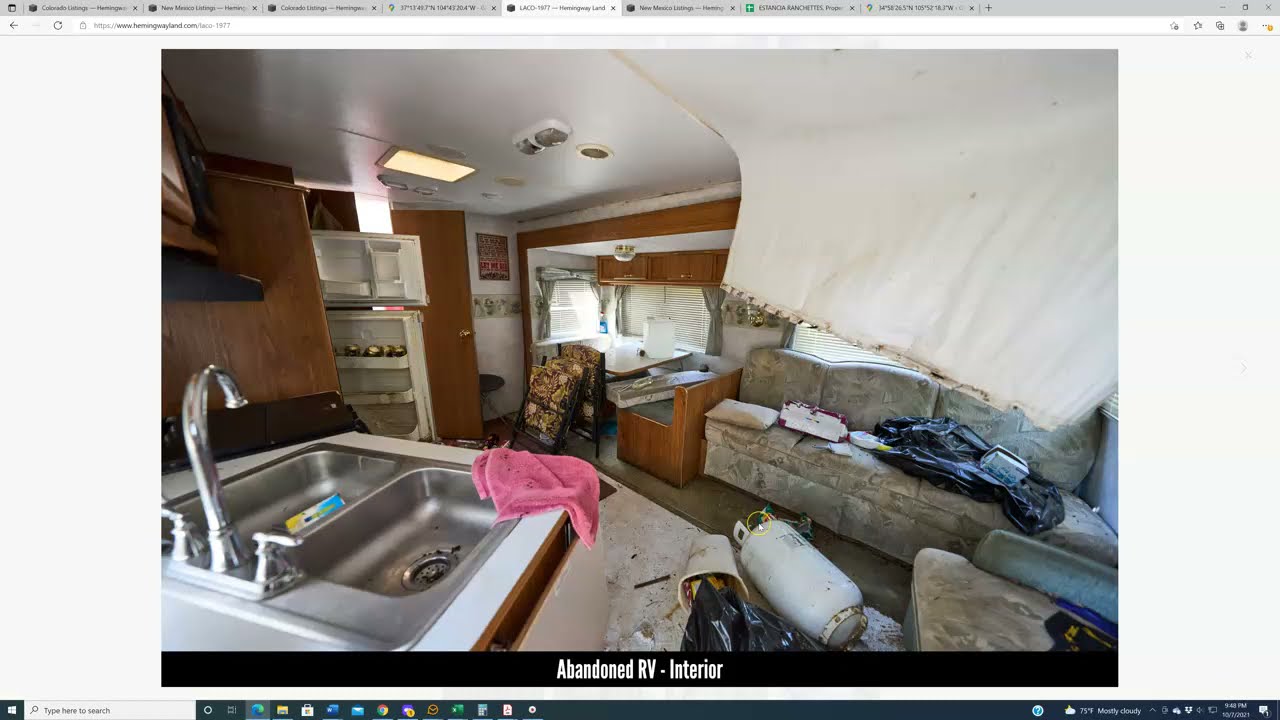In this detailed image, we are looking at a screenshot displayed on a computer monitor, evident from the visible headers, multiple tabs, and footers with various links at the top and bottom of the screen. Centered in the view is a snapshot labeled with a black banner in white text that reads "Abandoned RV Interior." The interior of the RV, seemingly afflicted by a hurricane, tornado, or storm, is in a state of significant disrepair. 

The roof's white lining is partially collapsed and curves downward over a long gray sofa positioned on the right side, which is cluttered with various debris, including a plastic garbage bag. Toward the right side, we also see two outdoor folding chairs leaning against each other, adding to the disorderly scene. Central to the composition is an empty but dirty kitchen sink decorated with a red or pink rag. To the left of it, the refrigerator stands with its top and bottom doors ajar, exposing its neglected state. Also near the center, a propane tank (or possibly a water heater) lies on its side, with an overturned garbage can nearby.

On the left, adjacent to the refrigerator, there is an eating area covered in miscellaneous junk, and a brown door with trimming can be observed. The overall atmosphere conveys abandonment and significant damage, capturing a moment frozen in disarray.